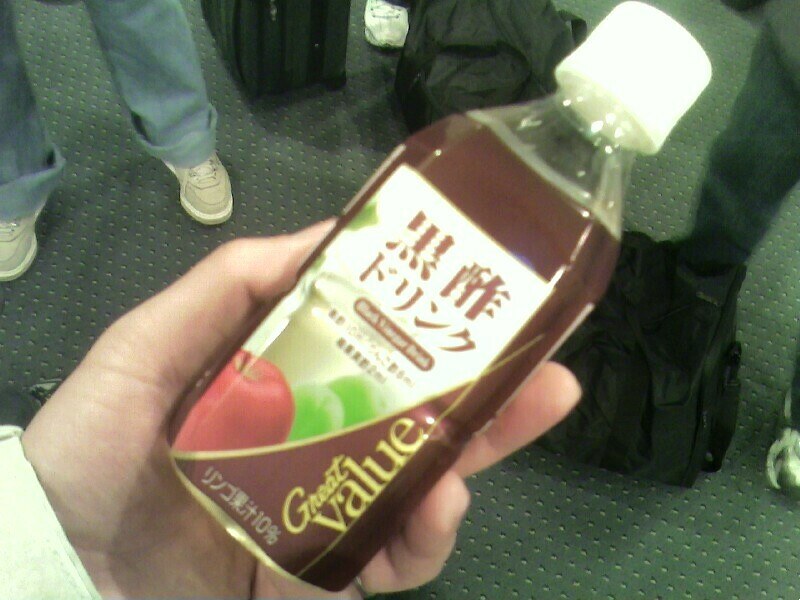This image features a clear plastic bottle with a white cap, held at an angle by a left hand, which appears to be a man's. The bottle has a brown label with white and brown lettering primarily in Japanese, except for "Great Value" written in English on the side. The label showcases a red apple and two green apples, suggesting the drink inside may be apple juice. The bottle's liquid appears brown. The background reveals a greenish-blue carpet with a subtle square pattern, along with multiple travelers' legs and feet, indicating a busy setting, possibly an airport. One person is wearing blue jeans and white shoes, while another's leg, clad in black pants, is visible next to a black tote bag. Additional luggage and bags are scattered around, reinforcing the travel context.